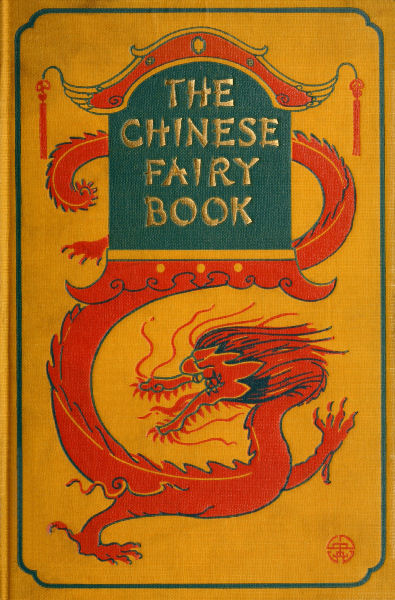This is a vertically aligned rectangular image resembling a book cover. The background features a brownish-gold hue bordered by a dark green frame. At the top center is a dark green section with an arching top, containing the gold-printed title, "The Chinese Fairy Book." Extending from behind this green section, a red dragon curves through the cover in a backward 'S' shape, with its open mouth and fangs pointing towards the left at the bottom center. The dragon appears to be breathing fire. The cover’s design is further accentuated by subtle curved lines around the dragon, encapsulating the mythical essence and Chinese fairy tale theme.